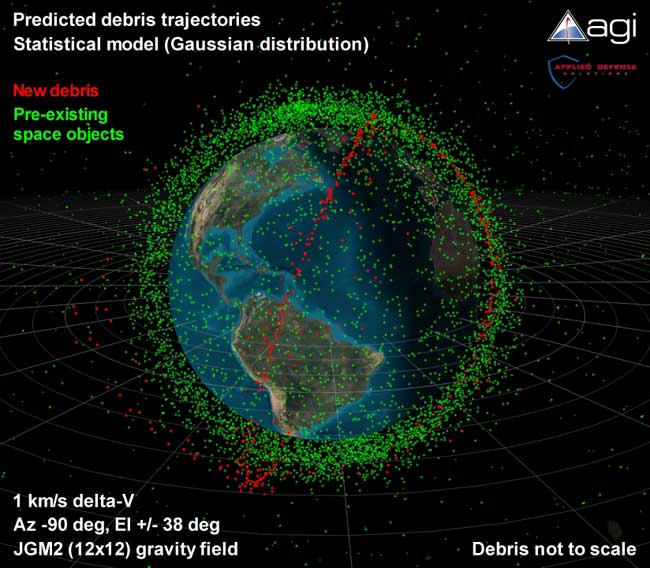This detailed image, likely a computer-generated render, depicts Earth surrounded by predicted space debris trajectories. The central visual shows Earth with the recognizable continents of North and South America in color, against a backdrop of space. Radiating out from Earth, green dots indicate pre-existing space objects, while red dots represent new debris. Labeled grids and statistical models, presented with a Gaussian distribution, envelope the Earth, illustrating the spread and density of these objects.

The image is bordered by informative text: in the upper right-hand corner, the logo and name “AGI Applied Defense” can be seen, suggesting the origin of the study. The title "Predicted Debris Trajectories Statistical Model Gaussian Distribution" stands out prominently. Additional text in red identifies "New Debris," while green text denotes "Pre-Existing Space Objects." Mathematical annotations and equations like "Delta V, AC-90, DLG, EI, ±38° G, JGM2 12x12 Gravity Field" appear around the image, underpinning the scientific basis of the model.

In the background, a black space field accentuates the bright green and red dots. The blue sphere of Earth contrasts starkly with the dark surroundings, bringing focus to the planetary depiction. At the bottom right-hand corner, a note clarifies that the debris is "not to scale," ensuring viewers understand the relative sizes and distributions presented.